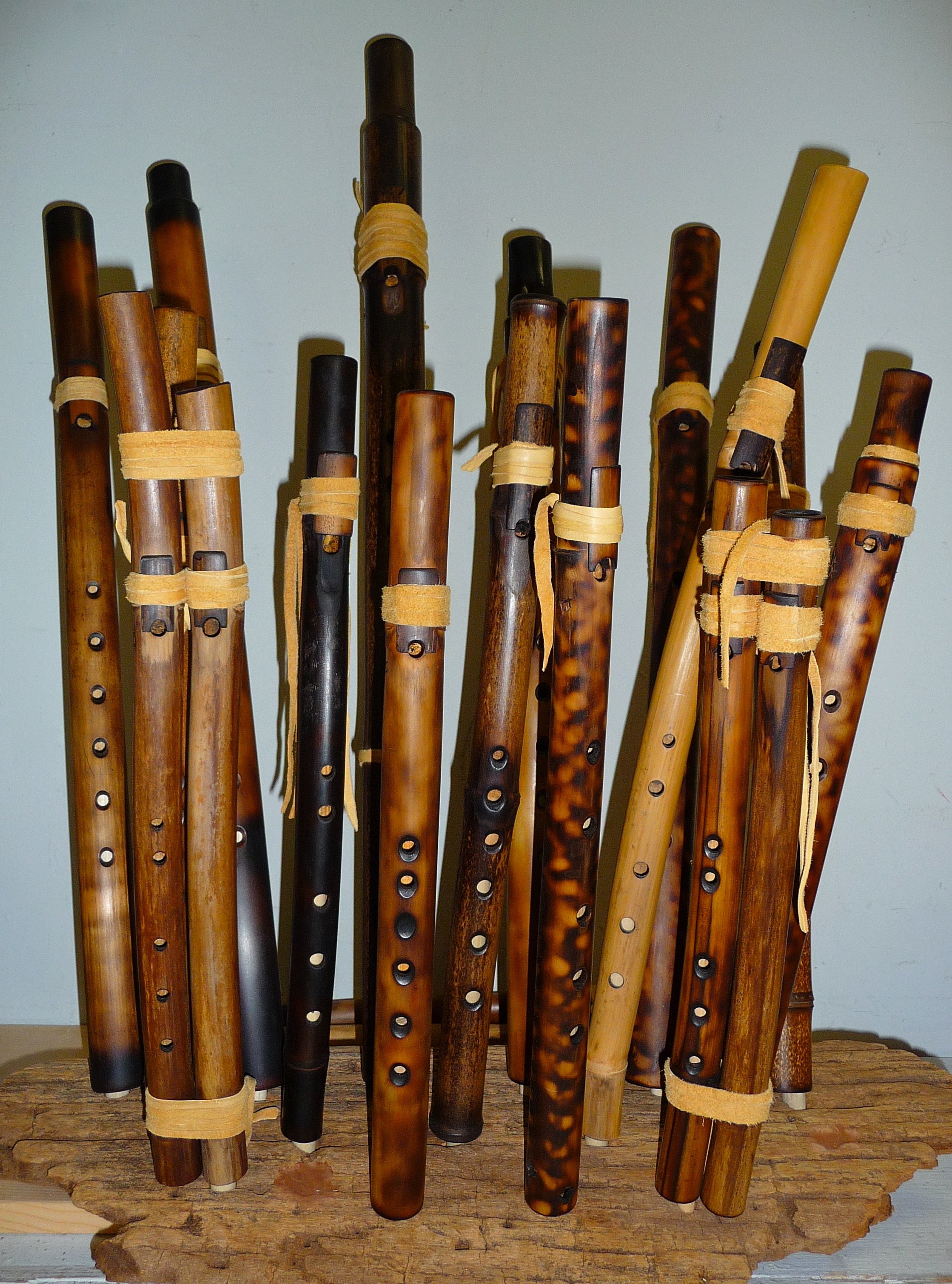The photograph captures a vertical arrangement of approximately twenty handcrafted wooden flutes displayed against a light blue or white background. These flutes, varying widely in color and pattern, rest on a rustic, irregularly-shaped wooden platform that seems to be cut directly from a tree stump. The flutes exhibit a range of natural wood finishes, including light brown, dark brown, near-black, and multicolored grains. Distinctly handcrafted, each flute features around six metal holes along its length and is adorned with bindings made from animal hide or a similar material. Some flutes are bound together in pairs, enhancing their visual variety and adding a unique element to the display. The overall composition and the rich textures of the wood make the collection not only functional as musical instruments but also an intriguing piece of art.